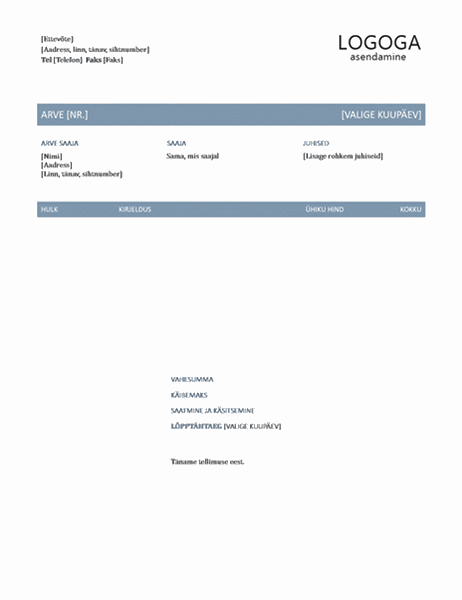The image depicts a screenshot of an invoice or billing statement with a white background and no border. The company name, "Logoga Acetamine," is prominently displayed in black lettering in the upper right corner. In the upper left corner, there is a section with black text intended for the recipient's name, address, and telephone number. Below this section, a thick blue or light gray banner spans the width of the image, featuring white lettering that appears to say "Arrive" followed by "(N-R)." This is mirrored across the left and right sides of the banner. Subsequent to this banner, there is a columnar arrangement of black and blue text providing detailed information, divided into sections for the recipient’s information on the left, and additional details in the middle and right columns. Another blue banner with white text is situated further down the page. Towards the bottom of the image, there is centrally aligned black lettering against a white background, with additional name and address details presented. The text throughout the invoice appears to be in a foreign language.